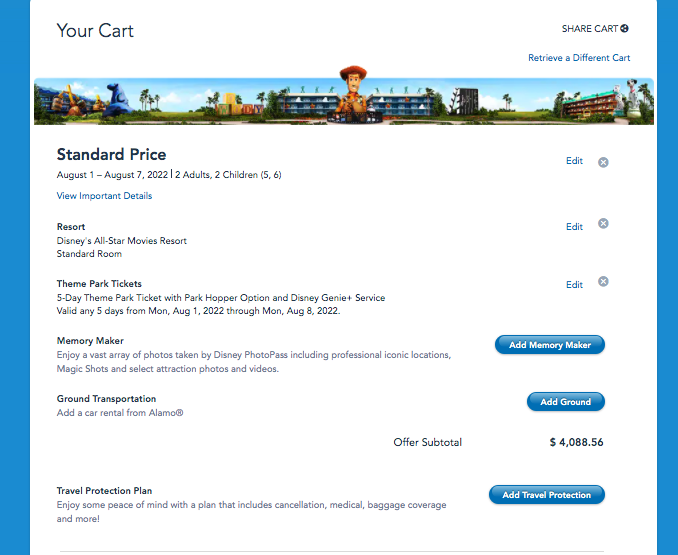The screenshot captures the shopping cart section of a predominantly white website, accented by thin blue margins on the left and right edges. At the top left, "Your Cart" is displayed in thin black text, while at the top right, smaller black text reads "Share Cart," followed by blue text offering the option to "Retrieve a Different Cart."

A prominent banner features various Disney Resort landmarks, with Woody the Cowboy from Toy Story smiling directly at the viewer from the center.

Three products fill the shopping cart:

1. **Resort Reservation**: 
   - Date Range: August 1st - August 7th, 2022
   - Guests: Two adults and two children (ages five and six)
   - Resort: Disney's All-Star Movies Resort, Standard Room
   - Additional Details: "View Important Details" link in blue text

2. **Theme Park Tickets**:
   - Type: Five-day Theme Park Ticket with Park Hopper Option and Disney Genie Plus Service
   - Validity: Any five days between August 1st, 2022, and August 8th, 2022

3. **Memory Maker** (Add-on, not yet activated): 
   - Description: Access to Disney PhotoPass, including professional photos, iconic locations, Magic Shots, and select attraction photos and videos
   - Action: A blue button labeled "Add Memory Maker"

Additionally, there is an option to add ground transportation from Alamo, with a blue button reading "Add Ground." 

On the right side, the subtotal is prominently displayed as $4,088.56.

At the very bottom, there's a mention of a "Travel Protection Plan," offering cancellation, medical, and baggage coverage. A blue button invites users to "Add Travel Protection."